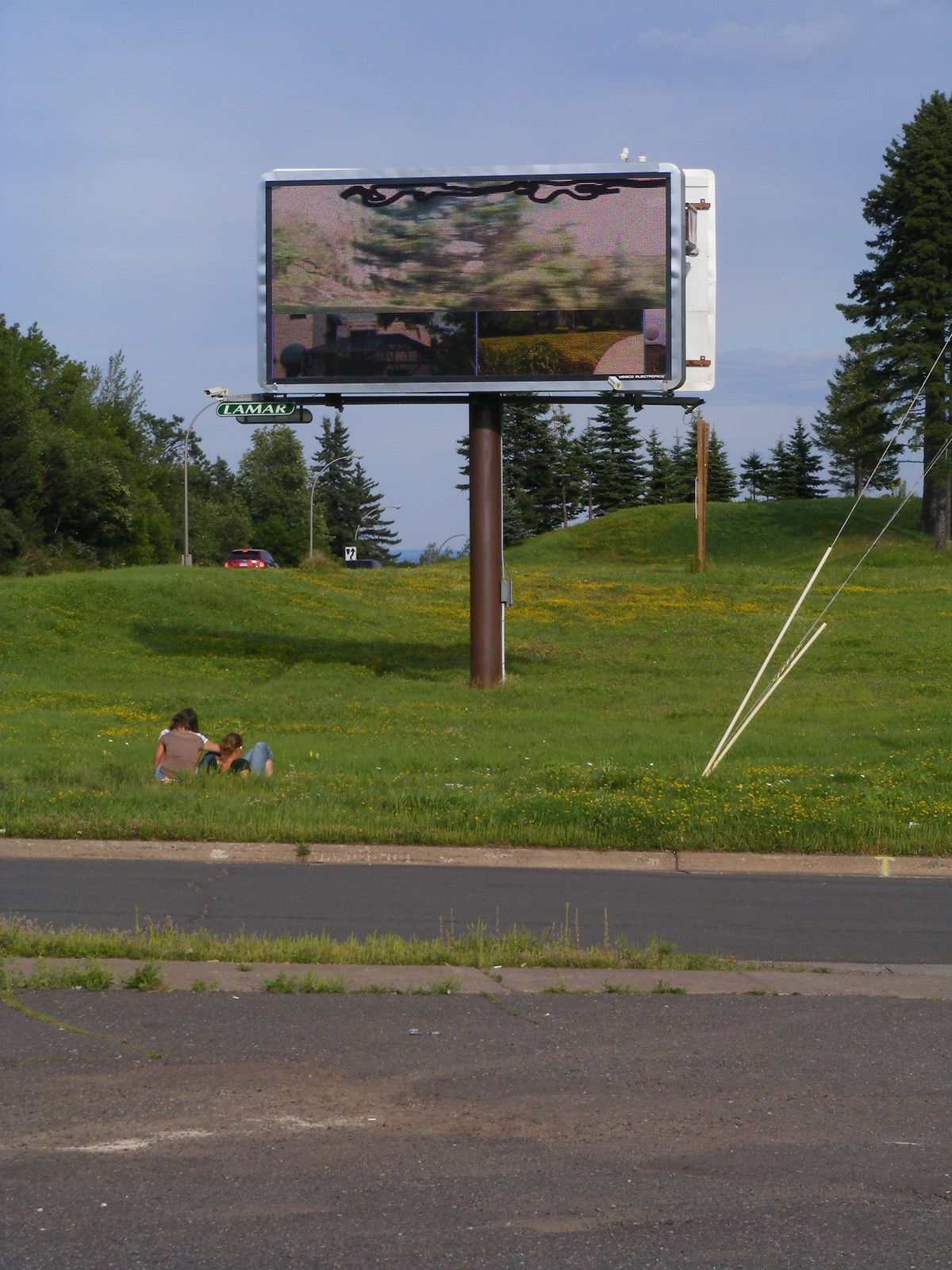The image depicts a daytime scene at a location resembling a drive-in theater, although it features a unique setup. At the forefront of the image is a parking lot, followed by a small grassy island, and then more parking spaces. On the left side, there are two white poles from which cables ascend at an angle toward the left, although their connection point is unclear.

Dominating the center of the image is a large brown pole supporting a screen that appears to be divided into three sections. The top section displays black squiggly lines against the backdrop of tree images, while the bottom two sections resemble security camera footage, showing views of a front door and a walkway. The screen bears the label "Lamar" at its base in the bottom left corner, suggesting it might be an advertisement billboard rather than a typical drive-in screen.

In the background, a clear blue sky stretches down to a horizon marked by evergreen trees, forming a natural border on both the left and right sides of the frame. On the right side of the screen, a car is seen traveling up a roadway flanked by more trees and patches of grass.

Near the bottom right corner of the image, two people can be seen lying on the ground, gazing at the screen. One appears to be a girl wearing a black shirt and jeans, with her hair tied in a ponytail. The other, seemingly another girl, is dressed in a red shirt and blue jeans, sitting up slightly as they both focus on the screen's unusual display.